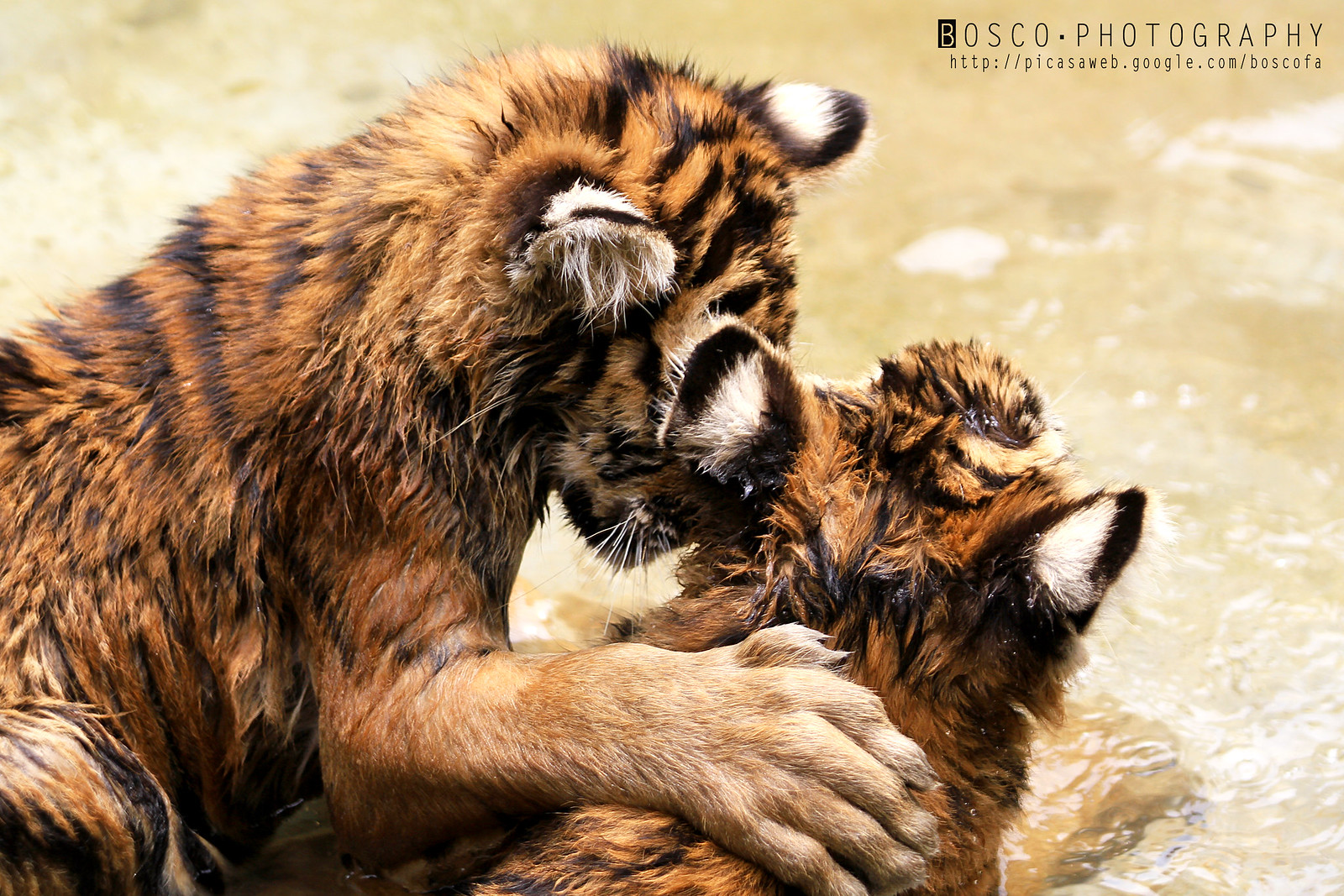The photograph captures an intimate moment between two wet tiger cubs playing in shallow, light brown water. The cub on the left, slightly larger, places its right paw on the back of the smaller cub on the right. The smaller cub is positioned almost fully with its back to the camera, while the larger cub is side-on, but its face is obscured by the other's ear. Both cubs exhibit matted, unkempt fur due to their frolic in the water. The clear, shallow water appears brownish through the translucence. Above the playful scene, the image is credited to Basco Photography, accompanied by a web address. The tigers display the classic orange, black, and white coloring typical of their species.